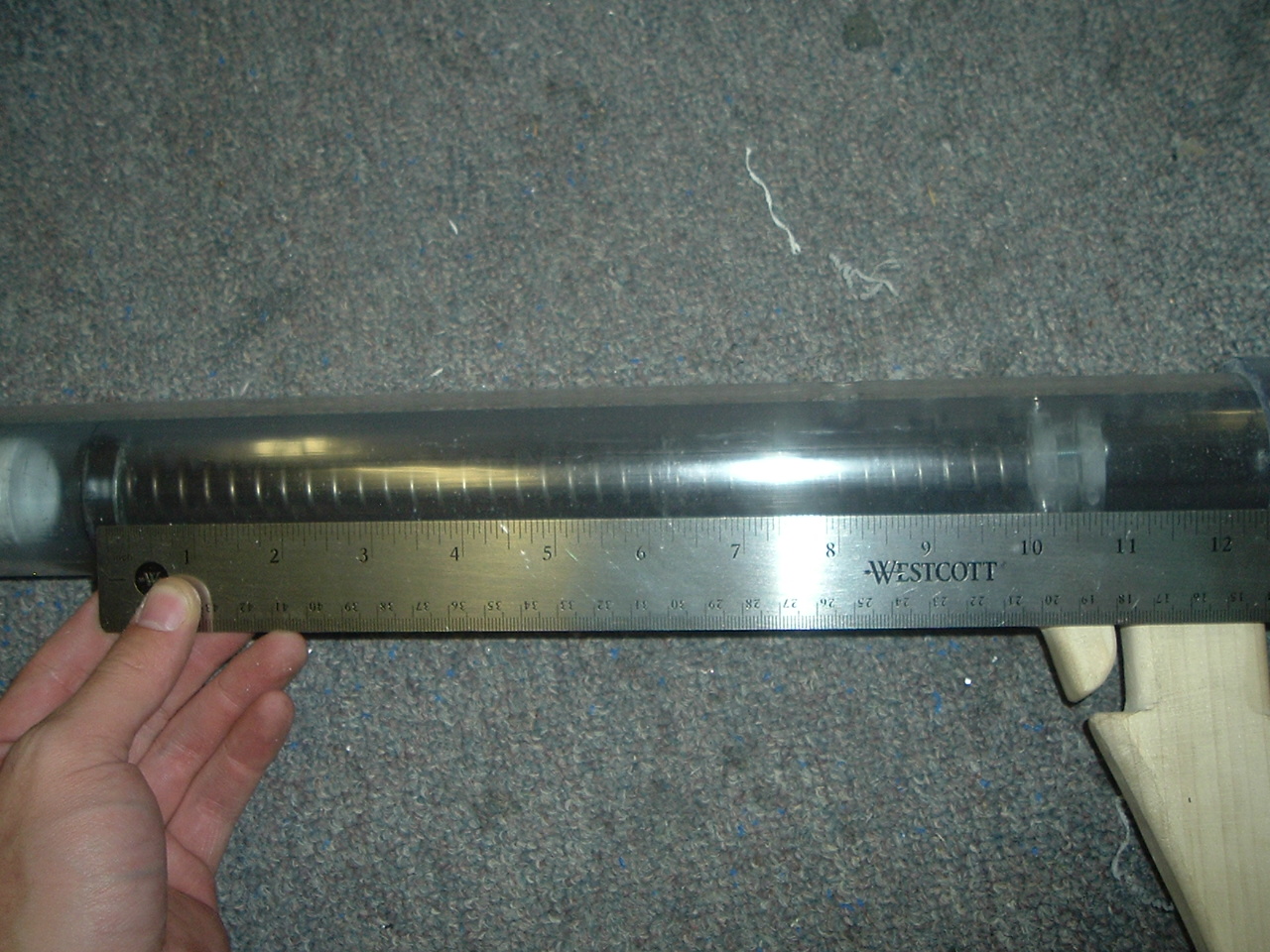In the image, a person is holding a 12-inch silver Westcott ruler, using their left hand, and the skin tone suggests they are white. The ruler is positioned against a transparent cylindrical object containing a coiled spring wrapped around a black tube. To the left of the tube, a white component resembling a trigger and handle suggests the object might be a paint gun. The setup is placed on a gray carpet, which appears unclean with a dark grayish pattern. Various items, including a white cord, are scattered on the carpet. A bright light intensely reflects off both the ruler and the transparent tube, highlighting the details in the image.